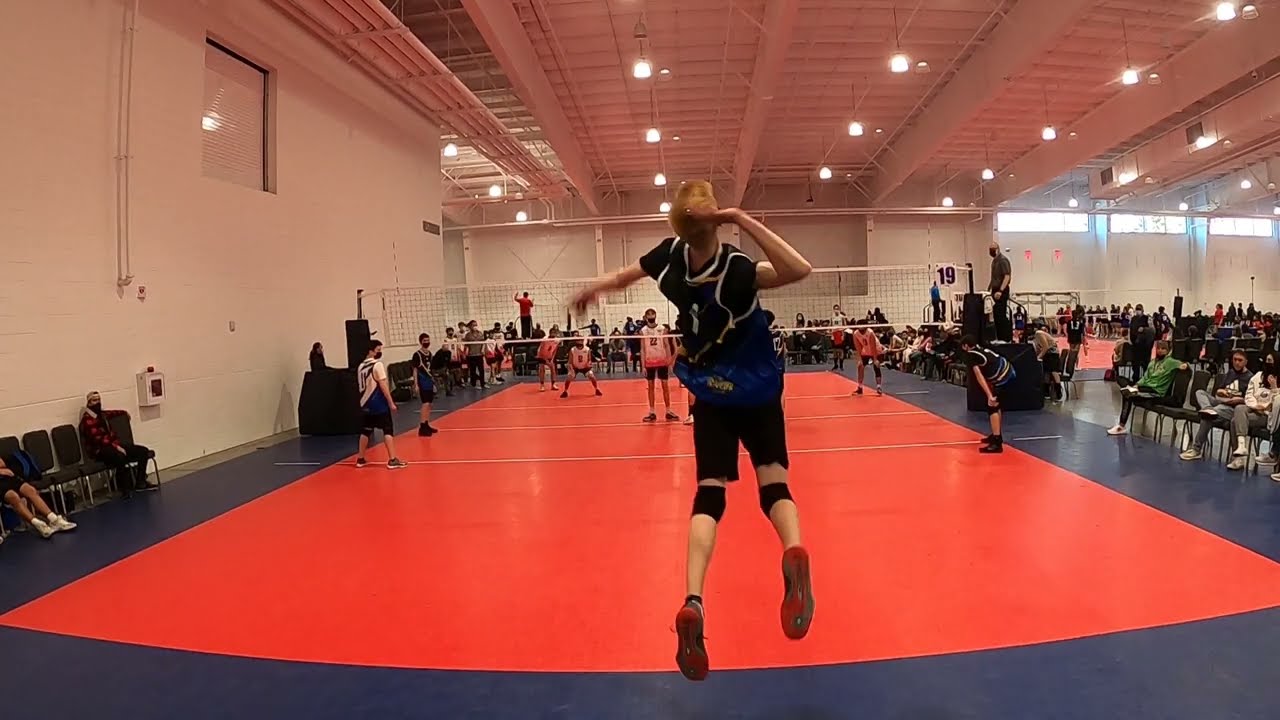The image captures an indoor volleyball game taking place in a large gymnasium. The scene is well-lit with globe-style orange lights hanging from the ceiling, which also features large white piping running both vertically and horizontally. The floor of the gymnasium is a hard surface painted as a sports court with a blue exterior trim and an orange center. Central to the image is a volleyball player with orangish-red hair, captured mid-jump with her right arm extended, aiming to strike the ball. To her right, a teammate bends over with hands on knees, while another stands upright. The opposing team is dressed in red and white jerseys with black pants, and numerous players can be seen scattered across both sides of the net.

Surrounding the court, there are black chairs occupied by spectators and possibly trainers or managers. Some spectators are also visible standing at the back of the gym. The gym's left wall is painted white and has a large window with white blinds. In one corner, two Caucasian men are seated together. Despite the presence of many details, the image contains no text. Overall, the setting is indicative of an active, indoor, nighttime volleyball game with engaging spectators and players.